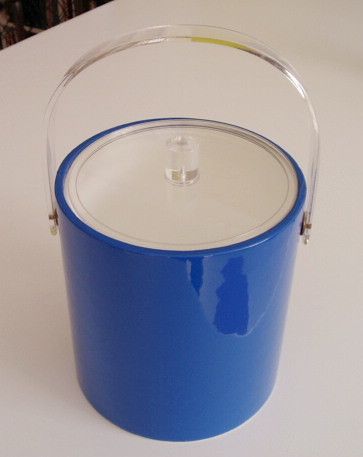The image shows a blue ice bucket, approximately the size and shape of a paint can, prominently occupying the white surface it rests on. The ice bucket features a white lid with a clear leucite knob extending from its center. Adjacent to this knob, a curved, clear leucite handle arches over the top of the lid, fully extended. The ice bucket is placed on a white surface, possibly covered by a tablecloth, with a small portion missing in the upper left corner. This isolated setting has no presence of people, buildings, or vehicles, and the ice bucket is the central focus of the photograph.